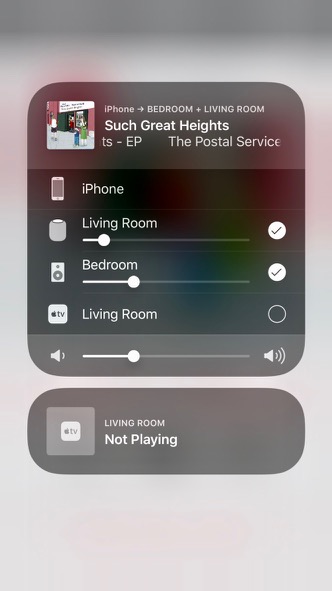The image depicts a cell phone screen showing the controls for Smart Home devices, focused on media playback through different speakers. 

At the top, the song "Such Great Heights" by The Postal Service is displayed as currently playing on the iPhone. Despite the iPhone being listed, there are no selectable options for it. Below, the controls for various rooms are shown:

- **Living Room**: The volume is set extremely low, indicated by the slider being positioned all the way to the left. The option is checked.
- **Bedroom**: The speaker here is set to a moderately higher volume compared to the Living Room, and this option is also checked.
- **Living Room** (listed again): This time, it is not checked.
  
Further down, there is an overall volume control set at approximately 30%. Below this control, a small bubble indicates "Living Room" is not playing. 

The background is a blurred or whited-out section, likely a zoomed-in portion of the album cover, making it indistinct and more of a backdrop. The interface elements, including the boxes and text, are rendered in black and gray with white writing, presenting a sleek, modern aesthetic.